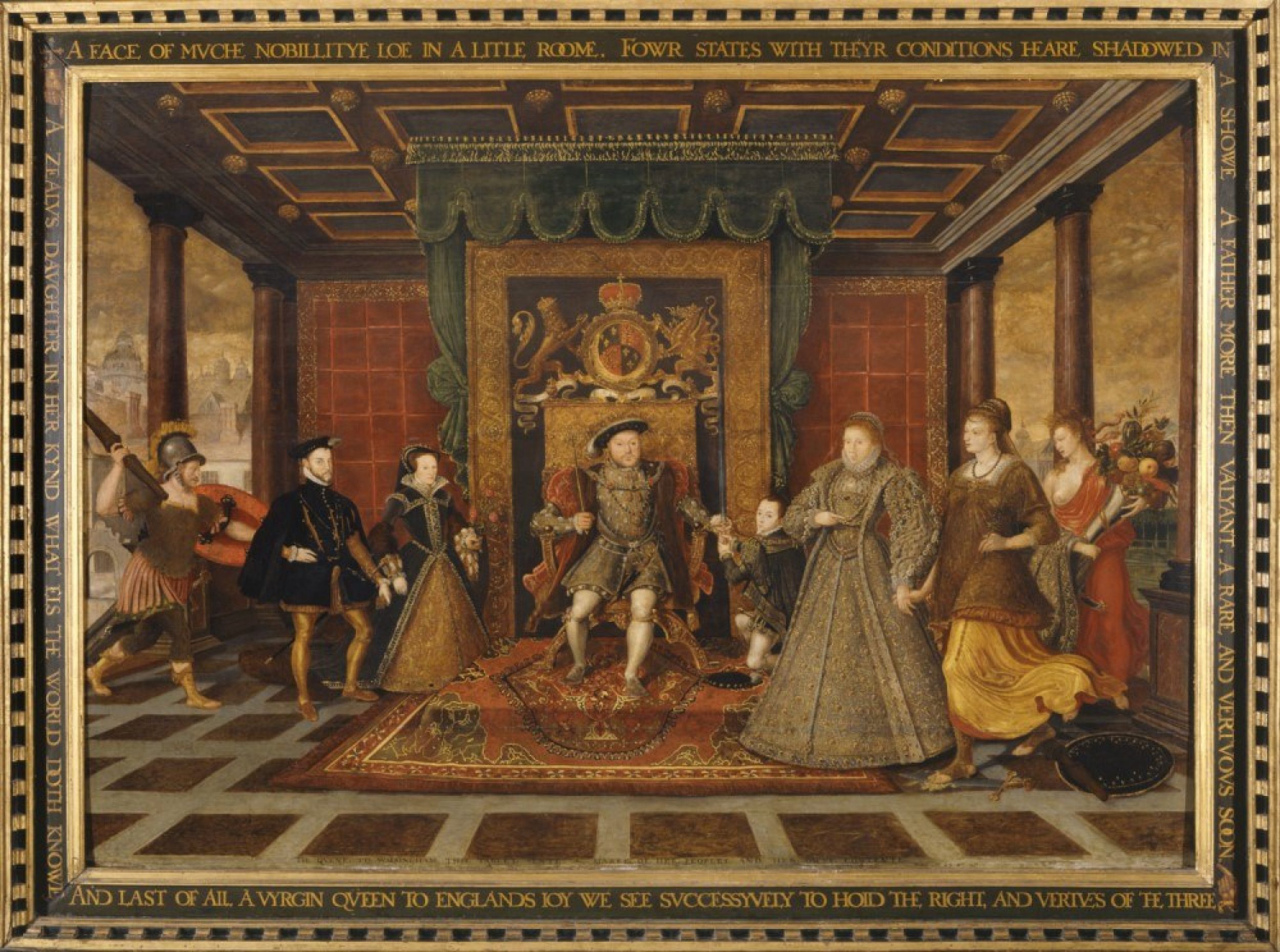The image is a horizontally aligned rectangular painting bordered by a gold frame adorned with black rectangles creating a pattern. At the top of the frame, it reads, "face of MVCHE nobility LOE in a little room. FOWR states with their conditions here shadowed." Further text along the sides and bottom of the frame includes a partially misspelled inscription: "and last of all a virgin queen to England's joy we see successfully to hold the right and verives of the three."

Set in a richly decorated room with a gold-toned background, the scene features a prominent figure, a king seated on a throne at the center. He is depicted with a thin build reminiscent of a stylized Henry VIII, wearing a black hat, dark brown and rust-colored clothing, and large puffy sleeves on his red coat. In front of him is an area rug. To the right of the king, a woman in a long, gold-colored gown, possibly the queen, stands elegantly.

The room is populated by several other figures. To the far right, a warrior with a metal helmet holds a standard in his right hand and a shield in his left. Next to him, a lady dressed in ornate black and gold attire is visible. On the far left, a well-dressed woman accompanied by two men stands; one of the men, potentially a soldier, wears a helmet and holds an indiscernible object, possibly a weapon or tool. Behind the central figures, another lady with exposed breast and simpler attire suggests varied status among the attendants.

The overall color palette of the painting includes browns, dull reds, golds, and muted tones, creating a classical and noble ambiance. Above the king’s head hangs a large coat of arms, adding to the regal setting. The intricate detailing and composition of the figures suggest a scene depicting courtly life and the hierarchy within.